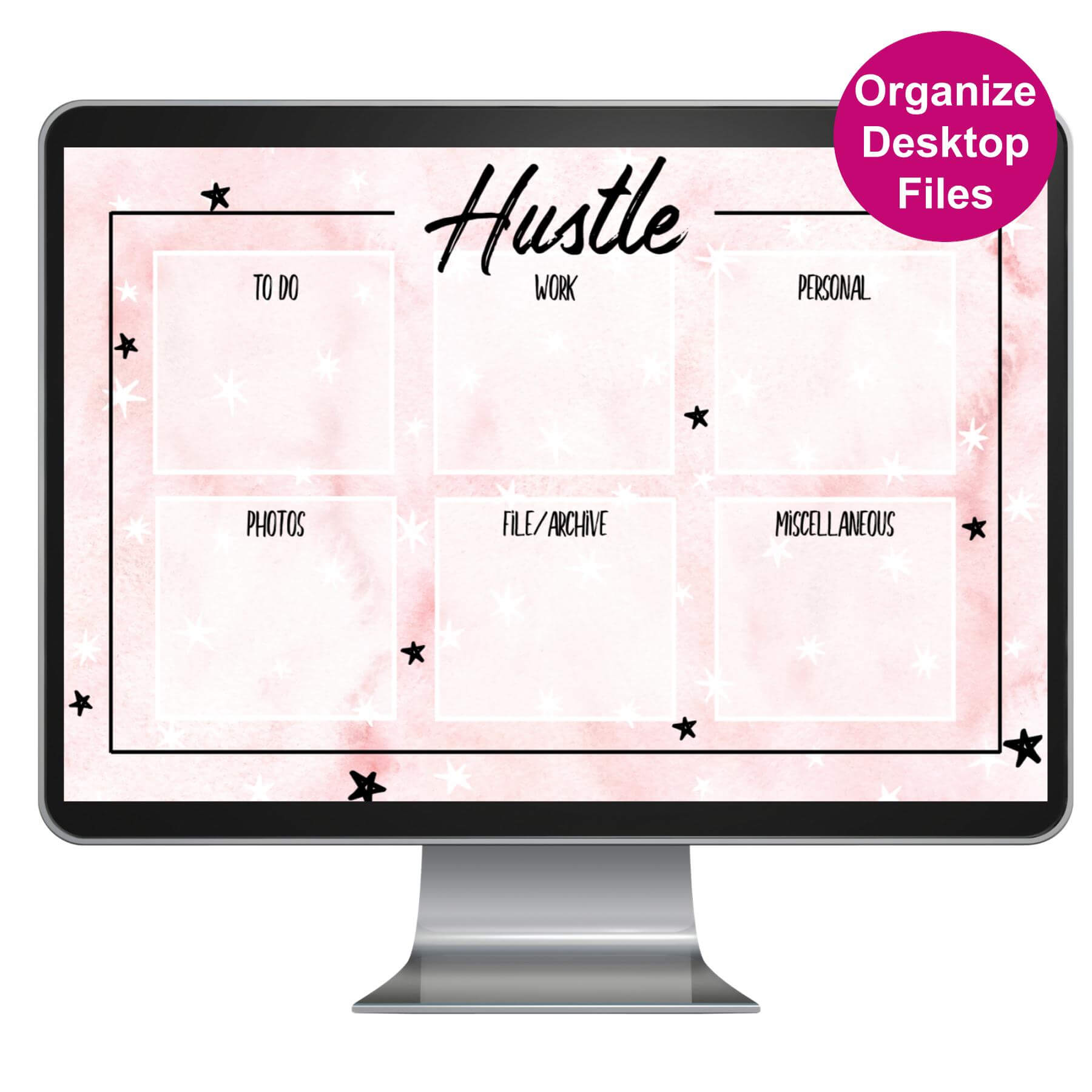This indoor color photograph showcases a sleek computer monitor with a modern silver base and a sturdy black border featuring rounded corners. The screen displays a pink background adorned with scattered black and white five-pointed stars, giving it a whimsical touch. Prominently at the top of the screen, in a distinctive black cursive font, is the word "Hustle."

Organizing the screen are two rows of three light pink boxes. The top row includes boxes labeled "To Do," "Work," and "Personal," while the bottom row features "Photos," "File Archive," and "Miscellaneous." Each box likely represents a section for organizing digital files, enhancing the usability of the computer workspace.

Adding to the visual appeal, the top right corner of the monitor displays a circular magenta badge with white text that reads "Organize Desktop Files." This detail indicates the photo's likely purpose as a promotional image for desktop organization software or an app, emphasizing a systematic and aesthetically pleasing way to keep one's computer files in order.